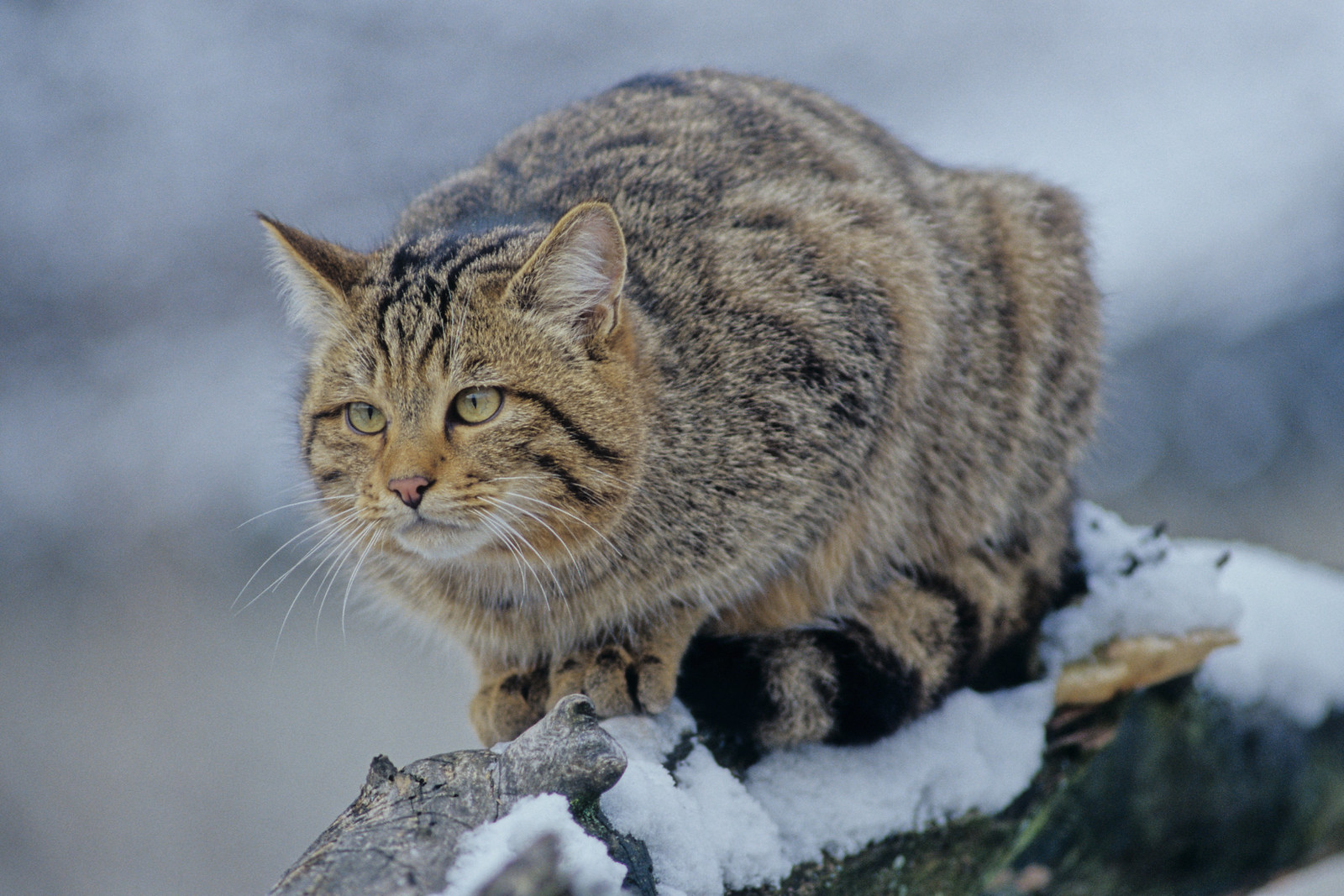In the center of this photograph stands a well-fed, thick tabby cat, perched atop what appears to be the snow-covered limb of a tree. The tabby displays distinct stripes on its forehead, cheeks, and tail, which is wrapped around its feet, possibly to keep warm amidst the snowy surroundings. The cat is intently staring at something off-camera with a determined expression. The background of the image is extremely blurry, making it difficult to discern specific details, but patches of white suggest a snowy, cold outdoor setting mid-winter. The overall color palette includes gray, brown, black, white, tan, and an almost illusionary touch of green.